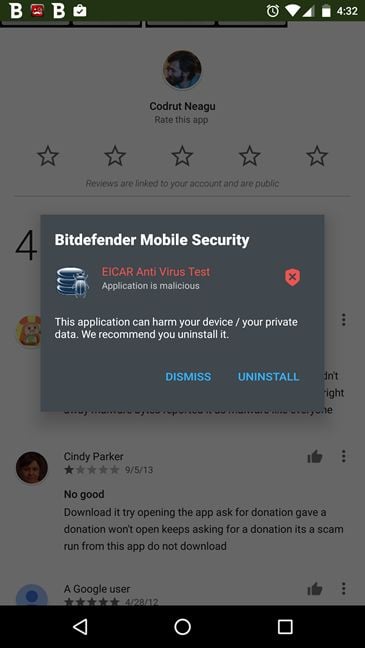Here's a detailed and cleaned-up caption for the described image:

---

This image depicts a mobile phone screen showcasing a security warning from the Bitdefender Mobile Security app. At the top of the screen, various status icons are displayed, including a symbol resembling the letter "B", a red box, another "B", a white briefcase icon, an alarm clock, a battery icon reading 43%, and the time, 4:32. 

The primary focus of the screen is a prominent gray pop-up notification from Bitdefender Mobile Security. In this notification, the word "Bitdefender" appears in white, followed by a red text stating "EICAR antivirus test." An icon of a red shield is displayed on the right. Below, it reads "Application is malicious" accompanied by a bug icon. The message continues with, "This application can harm your device/your private data. We recommend you uninstall it." Below this warning, two clickable options are visible in blue text: "Dismiss" and "Uninstall."

In the background of the pop-up, the screen is slightly grayed-out, showing an app review section. The title "Kodrat Negu" appears alongside his profile picture in a circular frame. He is about to rate the app, denoted by five empty stars. Below, a review by Cindy Parker is visible with a one-star rating. Her comment states: "No good. Downloaded it and tried to open. The app asked for a donation. Gave a donation, but it wouldn't open, keeps asking for a donation. It's a scam. Run from this app. Do not download."

---